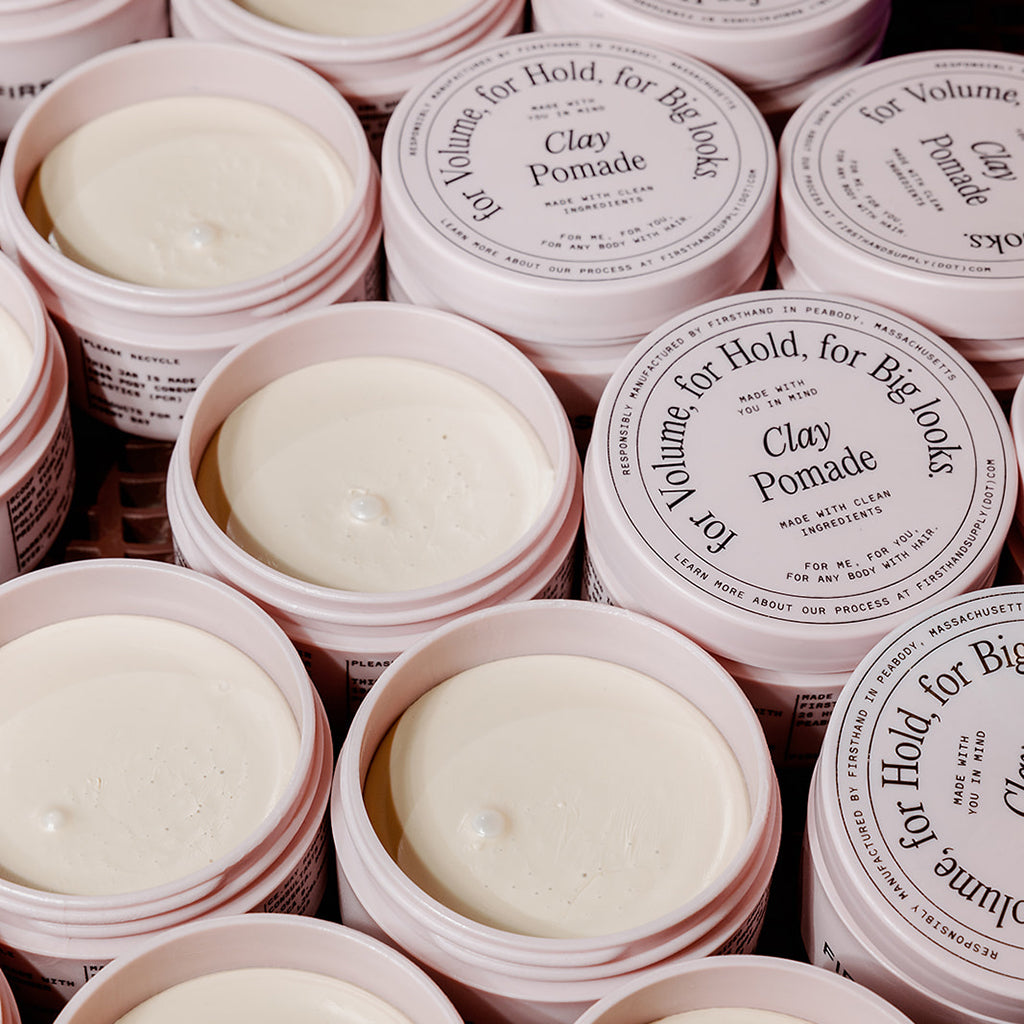This image displays an array of small, stubby pastel pink jars labeled "clay pomade." The jars, some with lids on and some with lids removed to reveal a white paste inside, are designed for hair styling, specifically for adding volume, hold, and creating big looks. The packaging features black text that reads: "For volume, for hold, for big looks." Additional details mention that the product is made with clean ingredients, with a message "made with you in mind." The rims of the jars also include more writing, and a website, firsthandsupply.com, is indicated for further information. The soft pastel pink hue of the jars contrasts with the white pomade and the black lettering, presenting a clean and modern aesthetic.